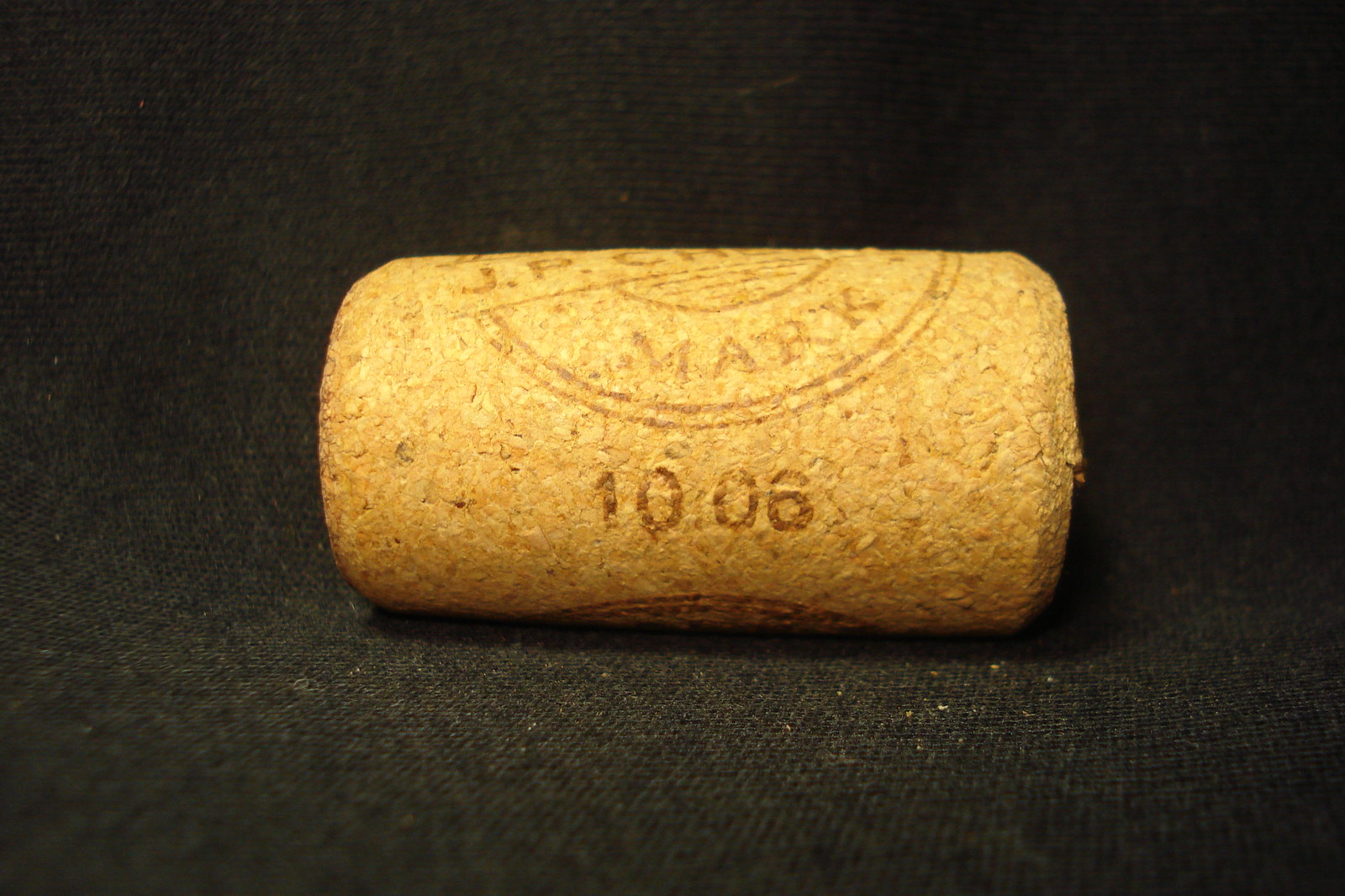This is a detailed close-up photograph of a wine cork, prominently placed on a black fabric background that provides a sharp contrast to the cork's tan, slightly yellowish-brown color. The spotlight centers on the cork, emphasizing its texture and details. The cork, robust and short, features a distinct emblem burned into the top, consisting of the names "JP" and "Mark" encircled, suggesting the maker's mark. Below this, the number "1006" is also seared into the cork with darker text. Little fragments of the cork can be seen scattered in front of it, adding to the authentic and tactile appearance of the scene. The image captures the cork in sharp focus against a dark, expansive backdrop, drawing attention to its intricately detailed surface and etched markings.